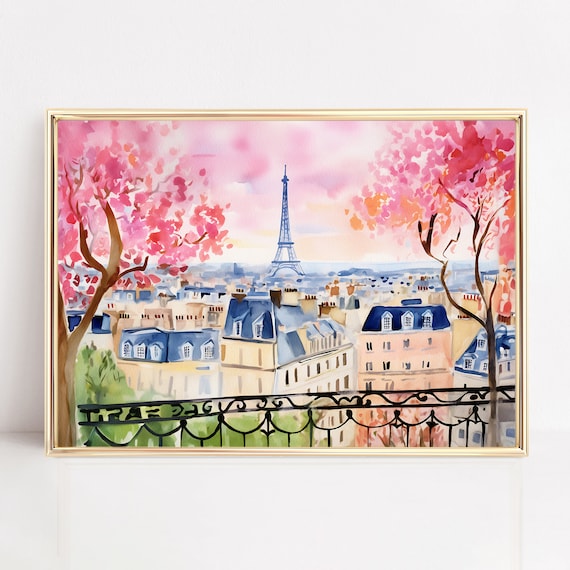This illustration or painting, possibly a watercolor in an ornate golden frame, depicts a picturesque scene of Paris. Central to the composition is a striking blue Eiffel Tower set against a sky tinged with pink and orange hues, suggesting a sunset. The foreground features a detailed black metal railing, evoking the feeling of viewing the scene from a balcony. On either side, blooming cherry blossom-like trees with pink and orange petals frame the image, blending seamlessly with the colorful sky. Below these vibrant trees are green foliage and quintessential Parisian buildings with yellowish-orange facades and distinctive blue roofs, detailed with numerous windows. This array of architectural and natural elements guides the eye naturally towards the iconic Eiffel Tower, making it the focal point of the painting. The entire artwork sits on a white background, enhancing its vivid colors and intricate details.